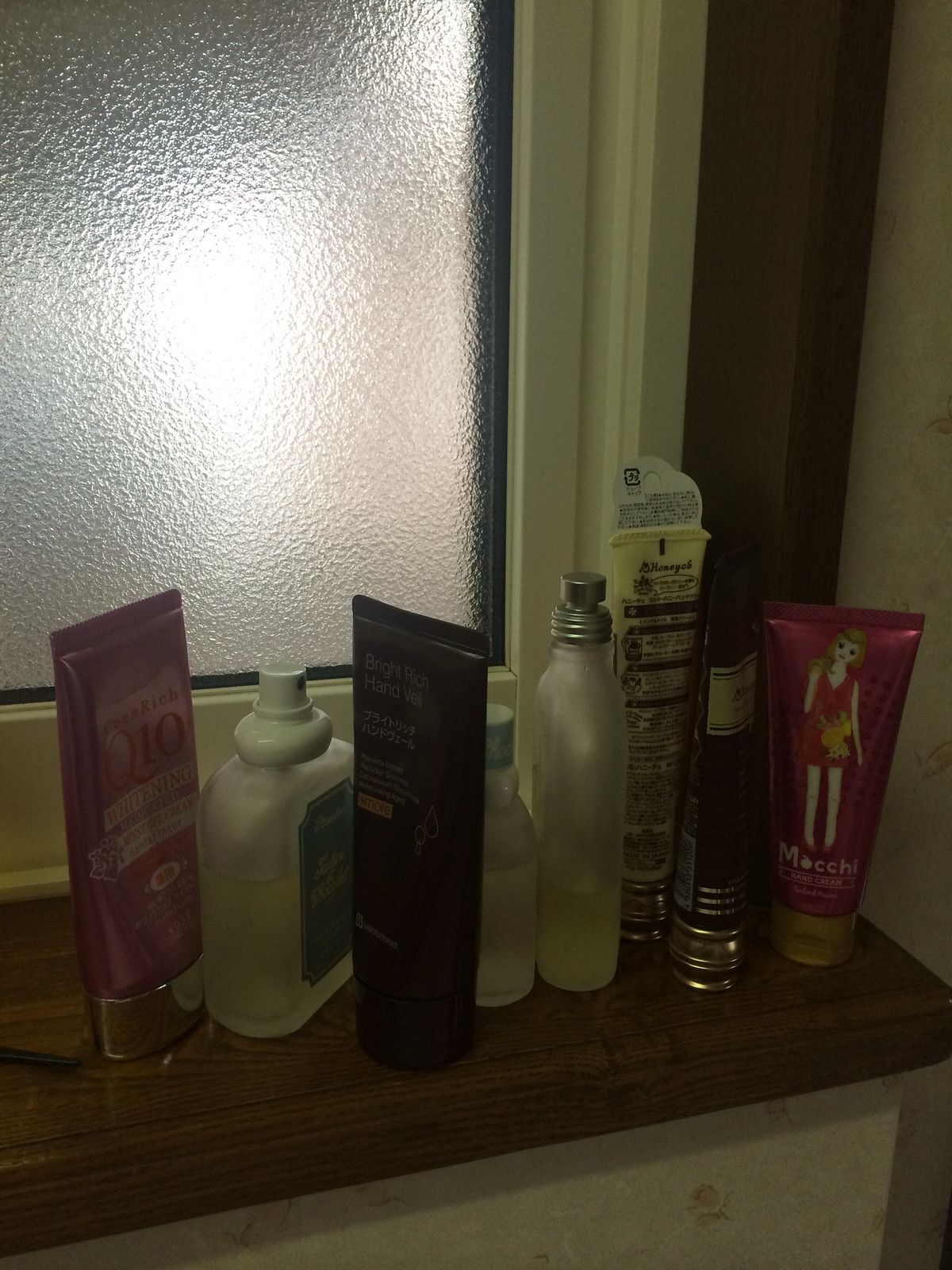This photorealistic image features a collection of eight various beauty products arranged on a dark brown, wooden ledge. The background includes frosted glass and sections of a white wall, with a prominent brown post attached to the ledge on the right side. The ledge spans diagonally from the top right to the lower left of the frame.

From left to right, the displayed items include:
1. A pink bottle standing on its reflective cap, featuring the label "Q10" with white designs.
2. A clear bottle with a white spray top, containing light yellow liquid, and a blue tag with white text.
3. A dark black bottle lying on a black cap, labeled "Bright Rich Hand Veil" in white writing.
4. A smaller clear bottle with a blue cap, also containing yellow liquid.
5. A larger clear bottle with a silver spray top.
6. A slender yellow bottle standing on a metallic cap, covered with extensive brown text on its back.
7. A dark-colored bottle on a gold cap, adorned with yellow designs on its front.
8. A pink bottle resting on a gold cap, displaying a cartoon of a woman in a pink dress with short brown hair, and labeled "Mochi" in white text.

While some bottles appear to be plastic and others glass, they collectively compose an assortment of lotions, sprays, and other beauty products, suggesting a setting likely within a bathroom or possibly a kitchen, given the functional and personal care nature of the items.